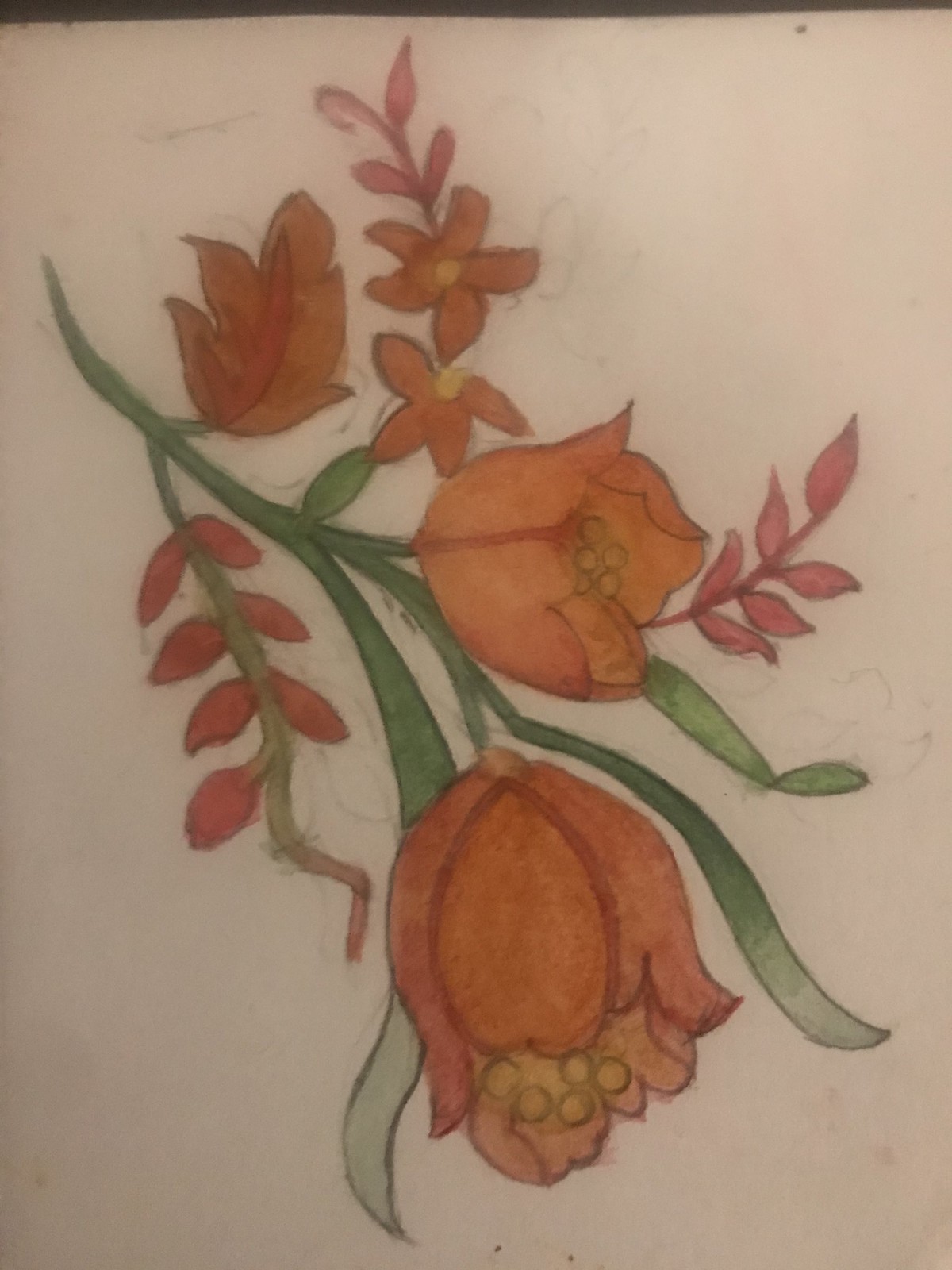This image captures a detailed hand-drawn artwork on white paper, which serves as the entire background. The drawing features an arrangement of orange tulips connected by a central green stem. The stem starts from the bottom of the image, pointing to the upper left corner, while the two main tulip bulbs face the bottom right corner. The larger bulb is located more towards the lower middle section of the image, and the smaller bulb is right above it, slightly towards the center. Accompanying the bulbs, there are several green and reddish-orange leaves branching off from the stem. Additionally, two smaller orange flowers are attached to these leaves. The artwork appears to be a mixed media piece, potentially combining watercolor and pencil, as evidenced by visible erased and redrawn lines. The overall arrangement of the flowers is tilted, making them appear upside-down in the image.